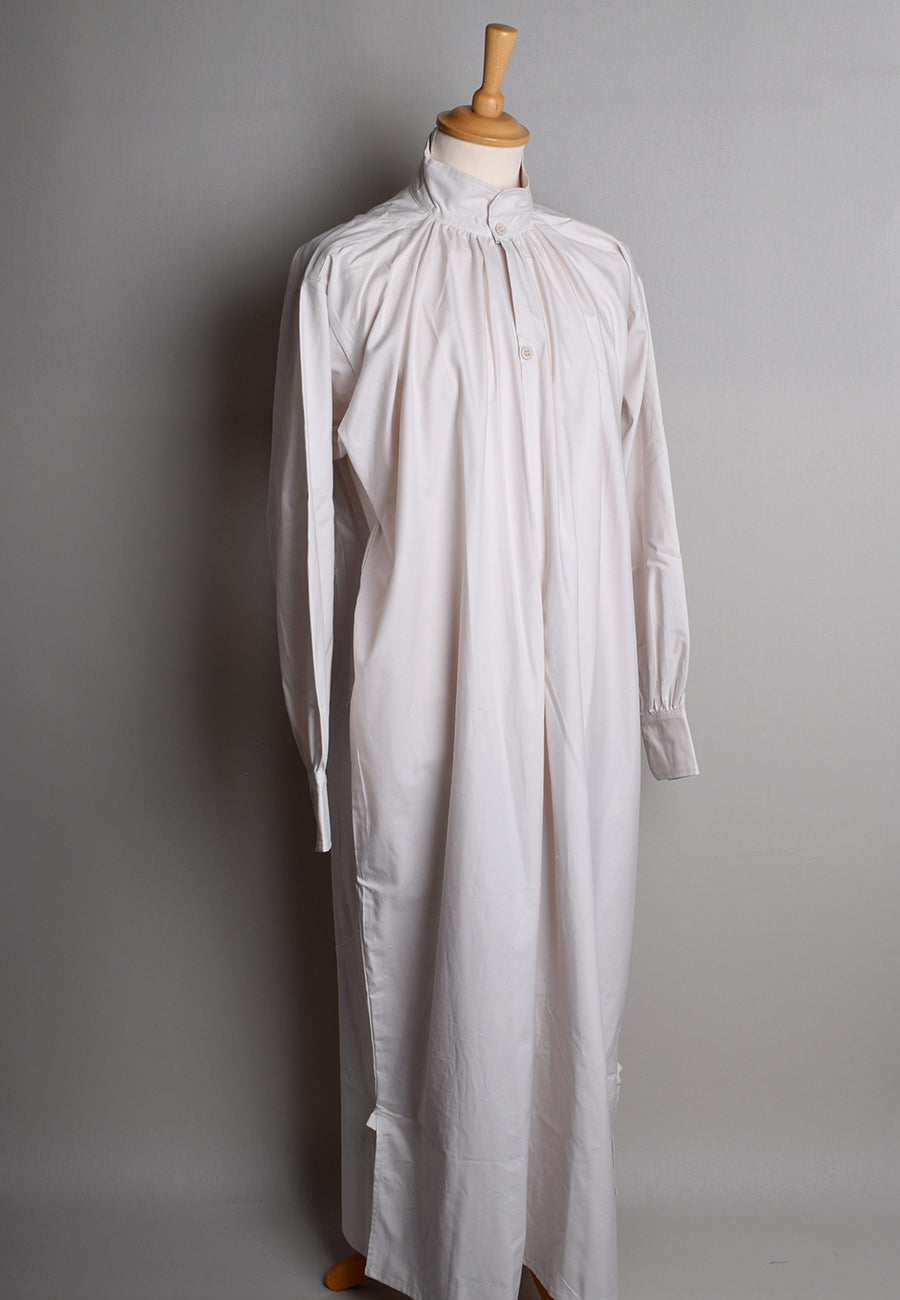The image depicts a white, long-sleeved gown draped over a headless dress dummy. The gown features a wide collar and is fastened with three buttons running from the collar down to the stomach. The sleeves are long and tapered at the wrists. A notable detail is the brown handle-like structure emerging from the neckline of the dress dummy, adding a curious element to its presentation. The gown also has a slit down one side, showcasing its elegant design. The primary colors in the image are white, with accents of brown and gray, contributing to the overall aesthetic.